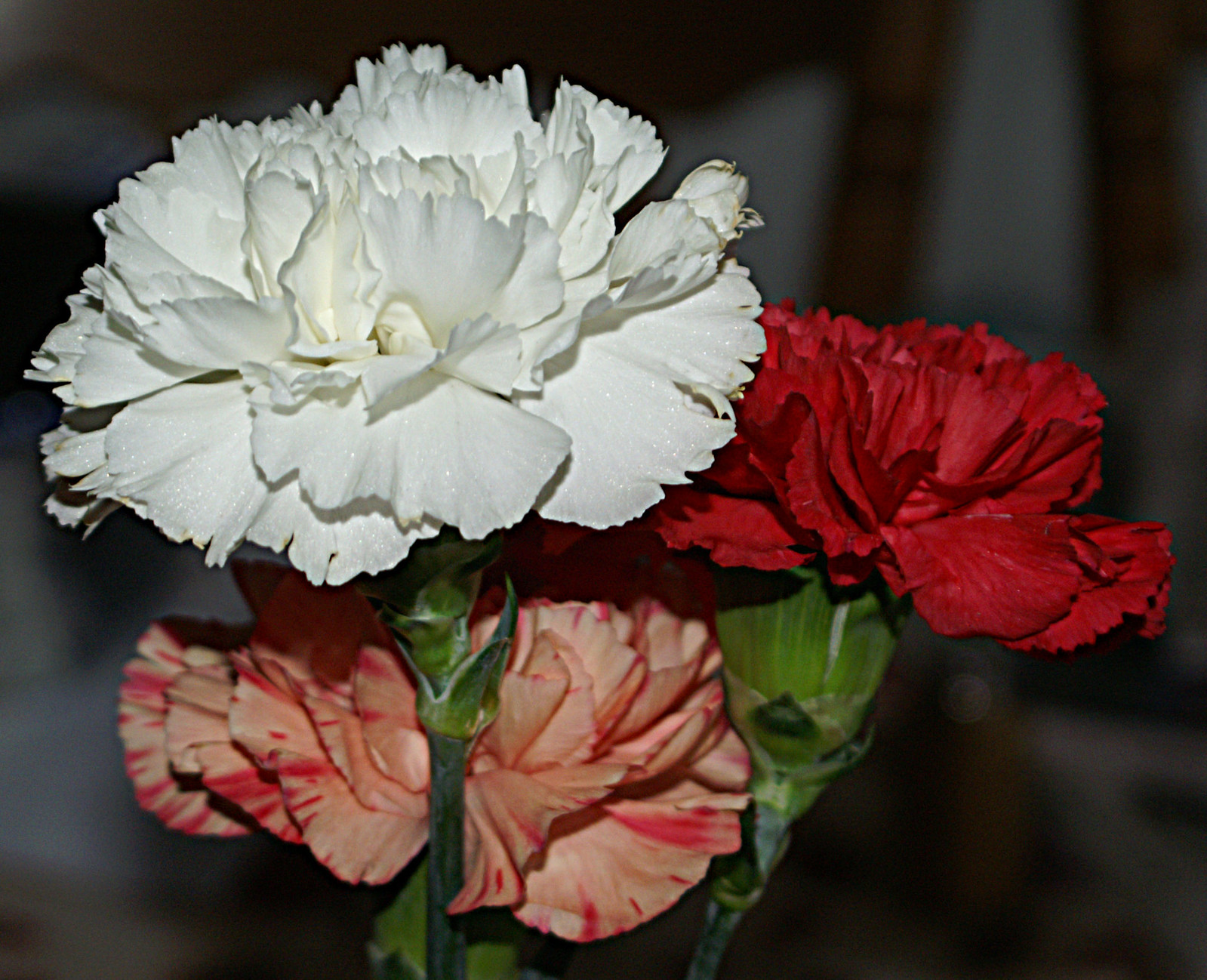This detailed close-up photograph captures a trio of flowers prominently centered in the image. The white flower, the largest and fullest of the three, is positioned in the top left and draws immediate attention. Slightly behind and to the right is a red flower with a rose-like appearance, standing out against the white bloom. Below the white flower and also somewhat recessed behind the red one, is a pink flower adorned with darker red stripes on its petals, giving it a unique blend of pink, peach, and red hues. All three flowers are connected by their green stems. The background is a blurry mix of dark gray and black, making it difficult to distinguish any specific details. However, some vague, rod-like structures are faintly visible, adding depth to the scene. The contrast between the brightly colored flowers and the muted, indistinct background emphasizes their vividness and intricate details.